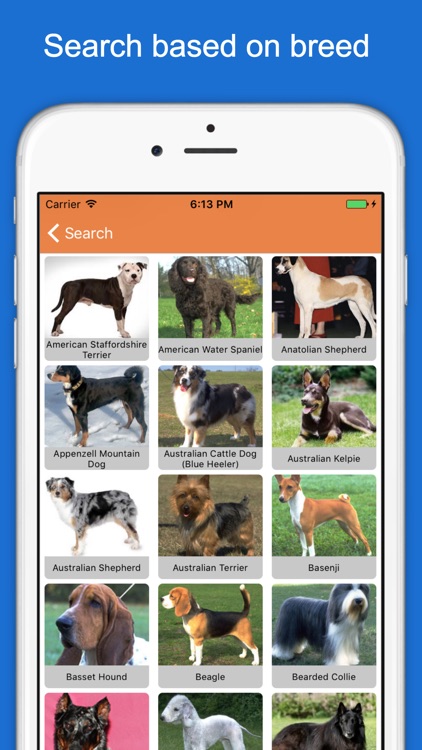A screenshot from a cellphone display showcasing a breed search feature for dogs. The interface has a soft royal blue background with a header at the top that reads "Search Based on Breed" in white text. Below the header sits a white cell phone with visible details indicating the battery is fully charged and the time displayed as 8:13 p.m. along with 6:13 p.m., and the network carrier information.

On the phone’s screen is an orange rectangular search bar located at the top. The main content area shows a grid of dog images organized in rows of three. Each image is labeled with a corresponding breed name. The first row features an American Staffordshire Terrier, an American Water Spaniel, and an Anatolian Shepherd. The second row displays an Appenzeller Mountain Dog, an Australian Cattle Dog (Blue Heeler), and an Australian Kelpie. The third row includes an Australian Shepherd, an Australian Terrier, and a Basenji. The fourth row contains a Basset Hound, a Beagle, and a Bearded Collie. The fifth row appears partially visible, showing images of three dogs whose breed names are not entirely displayed.